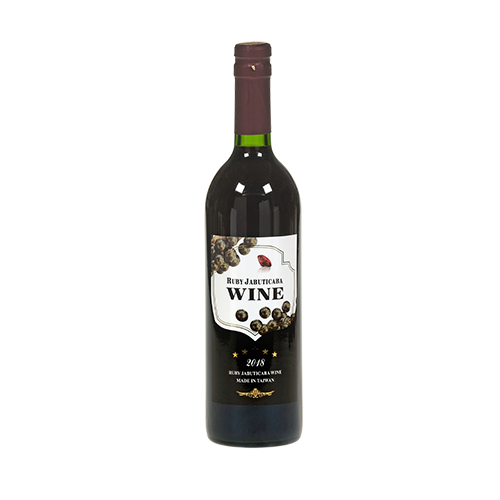This detailed photograph showcases a bottle of wine against a stark white background. The bottle, likely made of dark glass with a brownish hue, features a non-twist cap that necessitates a bottle opener. The neck and the cap are wrapped in a rich, dark burgundy sleeve. The primary label, with a white background and black bottom, displays the wine's name, although it is partially legible as "J-A-B-U-T-I-C-A-R-A Wine." This region of the label also includes dark grape illustrations. Below the central text, the vintage year "2018" is clearly printed. Adorning the label are four gold dots arranged in an arch, situated above a golden bird motif and some additional, unreadable text. The bottle reflects light distinctly, with two white light squares on the main body and two circular reflections near the bottle’s neck.